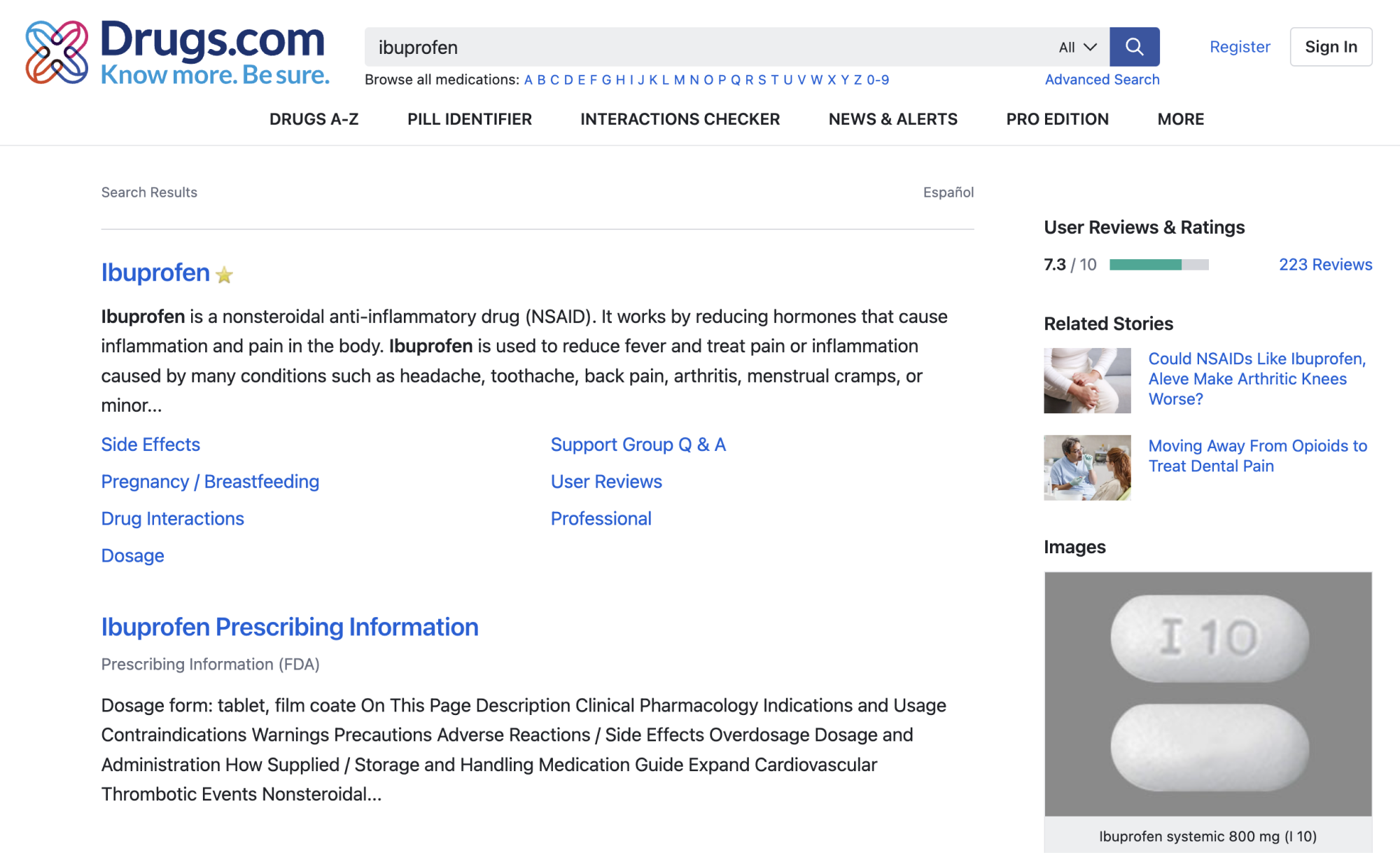The image features a screenshot of the website Drugs.com. Prominently displayed in the search field is the term "ibuprofen." The website's navigation menu includes options such as "Browse All Medications," "Drugs A-Z," "Pill Identifier," "Interactions Checker," "News and Alerts," "Pro Edition," and "More." The search results page provides detailed information on ibuprofen, describing it as a non-steroidal anti-inflammatory drug (NSAID) that works by reducing hormones responsible for inflammation and pain. The text explains that ibuprofen is commonly used to reduce fever and treat pain or inflammation from conditions including headaches, toothaches, back pain, arthritis, and menstrual cramps. Additional sections cover pregnancy and breastfeeding considerations, potential drug interactions, recommended dosages, support groups, Q&A, user reviews, professional advice, and prescribing information specifically for tablet dosages.